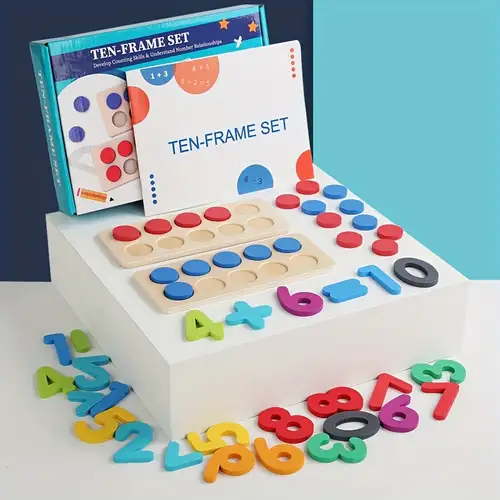In this photograph, we see an educational toy known as the 10 Frame Set, designed to develop counting skills and number relationships. The set includes an assortment of components arrayed on an elevated white surface against a contrasting background of dark and light blue. Central to the display are two wooden trays, each featuring two rows of five circular notches designed to hold small circular disks. The disks, colored in blue and red, are arranged to demonstrate basic arithmetic: one tray has four red disks and the other has five blue disks in the top row and one blue disk in the bottom row. Additionally, the setup includes colorful plastic numbers and mathematical symbols such as plus and equals signs, with "4 + 6 = 10" prominently featured.

Also visible in the image are various other multicolored number pieces scattered around, providing a vibrant and engaging visual. The box for the 10 Frame Set and its instruction manual can be seen positioned on the elevated surface. The overall arrangement showcases the educational value of the set, which is particularly useful for young children or beginners learning foundational math skills in a visually stimulating way.